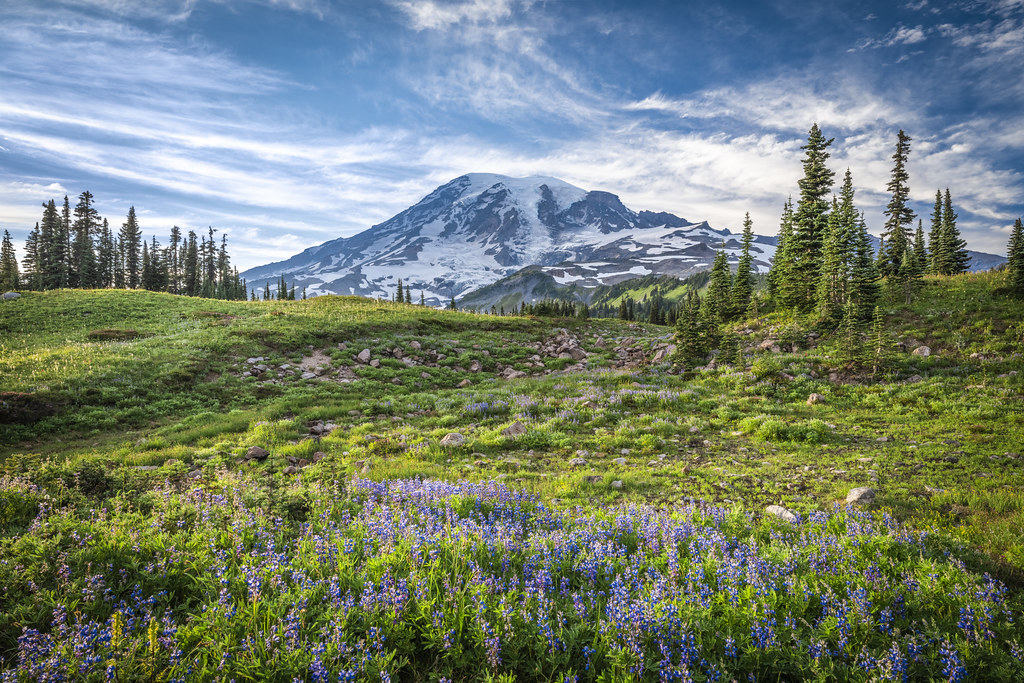This vibrant landscape photograph showcases a scenic meadow in what could be a Swiss alpine setting, reminiscent of scenes from "The Sound of Music." The image features a serene field carpeted in lush, newly-sprung greenery, dotted with small rocks and a variety of wildflowers, predominantly purple heather or lavender blossoms, which embellish the foreground. To the sides of the meadow, clusters of verdant pine trees provide a rich green frame, with their bright foliage standing out against the landscape. The background is dominated by a looming snow-covered mountain, its stark contrasts of white and gray ice symbolizing a chillier altitude. Above, a deep blue sky is streaked with dramatic, flowing mare's tail clouds, indicating a potential shift in weather. The overall composition harmonizes the vibrant yellow-greens of the meadow with the cool blues and grays of the mountain and sky, evoking a picturesque and tranquil atmosphere, perfect for a travel advertisement enticing visitors to this breathtaking location.